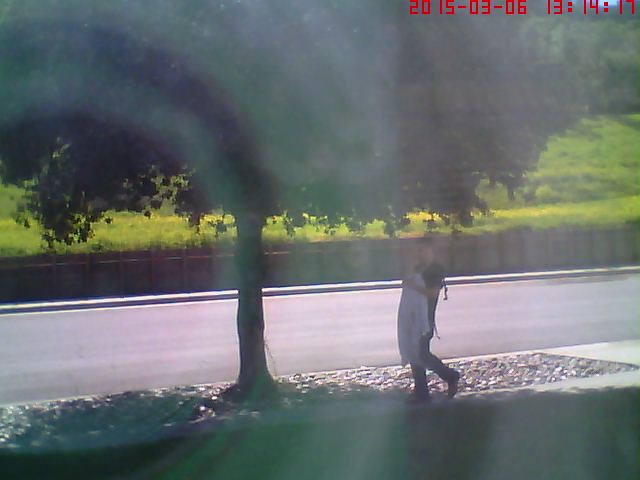This rectangular, landscape-oriented photograph, timestamped "2015-03-06 13:14:17" in red font in the top-right corner, captures a serene street scene. A person walks leisurely along the sidewalk, viewed from a side angle, heading to the left. Dominating the foreground, a majestic dark brown tree stands sentinel, its roots surrounded by a scatter of rocks. Behind this natural emblem, a brown fence stretches horizontally, delineating the space between the sidewalk and a verdant expanse. Beyond the fence, a lush carpet of light green and yellow grass extends, hinting at the arrival of spring. The composition invokes a tranquil suburban moment, frozen in time.